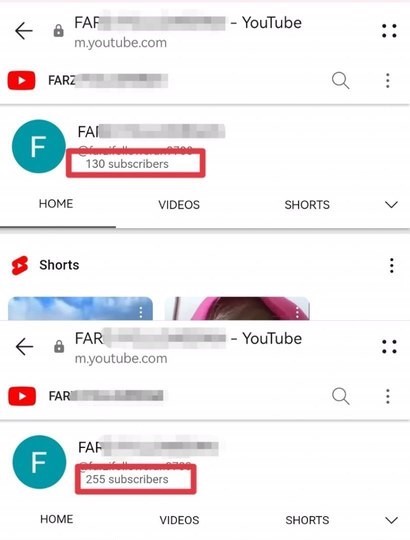This image consists of two vertically aligned screenshots from the YouTube app or website, each highlighting a specific YouTube channel using a red-bordered section to attract attention. 

The upper screenshot displays the YouTube channel page, though much of the channel’s title is obscured, showing only the partial name "Fars." The interface includes standard YouTube features such as a left-pointing arrow at the top left corner, likely for navigation, and a lock icon indicating the possibility of a private account. Below these icons, the YouTube logo is visible. The channel name appears again alongside the channel’s profile picture, and a search bar flanked by various menu icons crowns the top of the screen. Beneath the channel name, tabs for 'Home,' 'Videos,' and 'Shorts' are present, with a drop-down menu. Partial thumbnails of short videos can be seen towards the bottom of this screenshot. The focal point, marked by a red border, is the subscriber count, which stands at 130 subscribers.

The lower screenshot mirrors the layout of the upper one, displaying the same YouTube channel with identical icons and features in the same positions. However, the thumbnails for short videos are missing in this view. The most notable difference is again highlighted by the red-bordered section, which now shows the subscriber count increased to 255 subscribers.

Together, these screenshots illustrate a before-and-after comparison, emphasizing the growth in the channel's subscriber count.